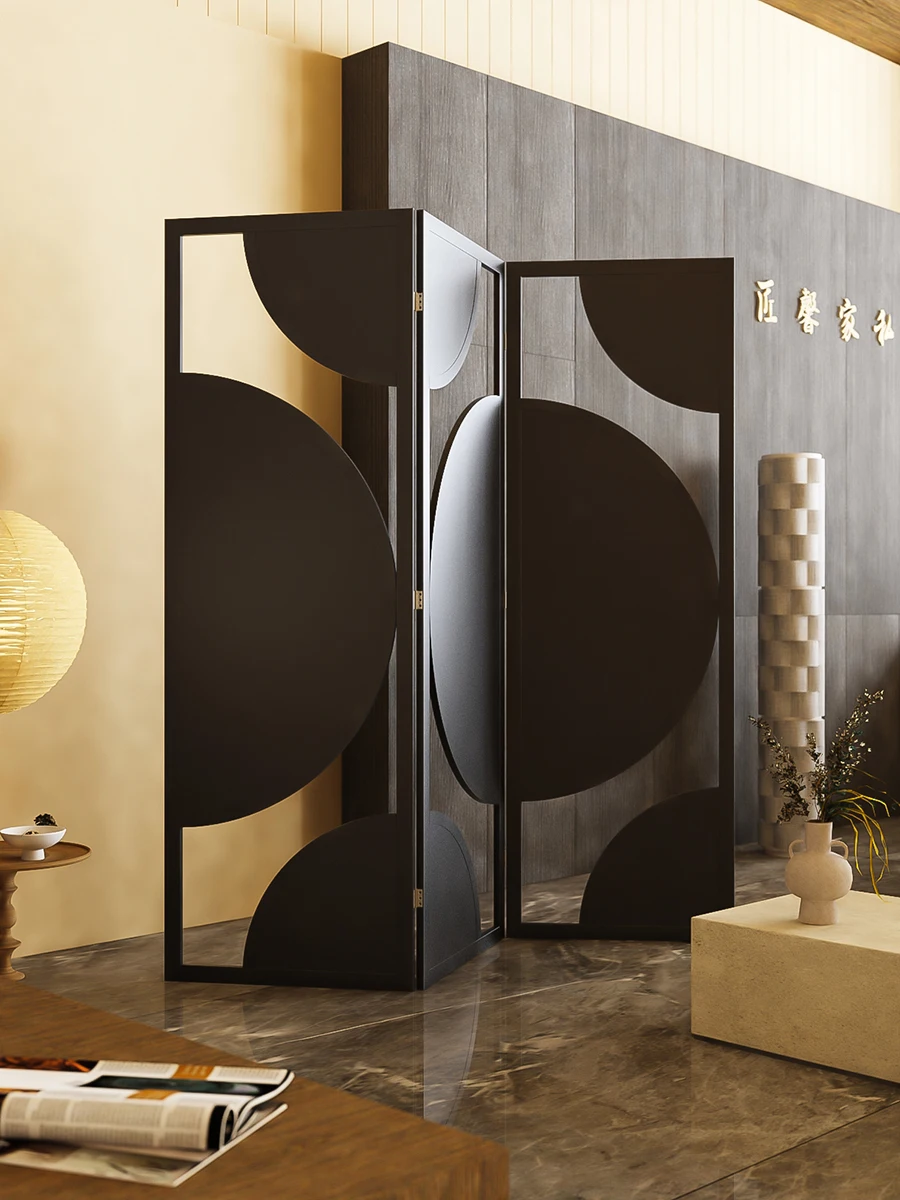The photograph captures the interior of a modern-designed room, possibly an Asian-themed restaurant or a stylishly furnished space. Dominating the scene is a decorative, black partition wall, with its clear sections framed by intricate half-circle designs, evoking the screens used in traditional dressing rooms. The wall behind this partition is adorned with golden Japanese or Chinese characters, standing out against a dark background. On the ground, a shiny, multi-toned marble floor reflects hues of tan, brown, and hints of orange, while a large wooden table in the bottom left holds an open magazine. Adjacent, a smaller round table supports a small white bowl, accompanied overhead by a yellowish, paper-style lantern that hints at Asian design elements. A two-handled clay vase, filled with long-stemmed flowers, adds a decorative touch in the foreground, and a white pillar stands to the right, complementing the beige walls and wooden paneling within the harmonious space.